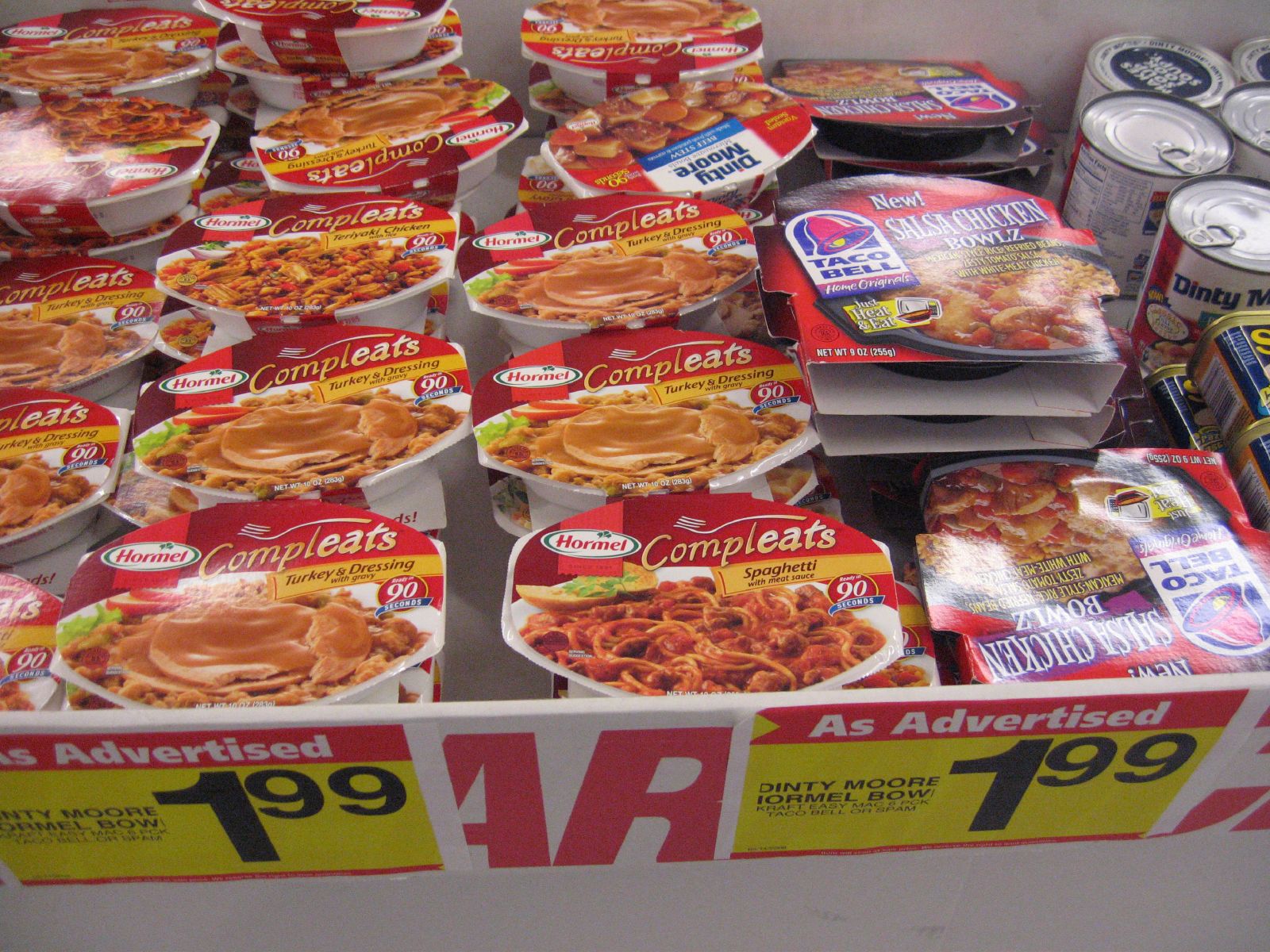The image captures a grocery store aisle featuring a prominent display of ready-to-eat meals and associated signage. The center of the display showcases two signs with a red strip at the top and a yellow background, boldly stating "as advertised" and "$1.99". These signs promote Dinty Moore Hormel Completes bowls, which include a variety of flavors like turkey and dressing, spaghetti with meat sauce, and teriyaki chicken. The bowls are designed for convenience, requiring only 90 seconds in the microwave to heat up. 

To the right of these bowls, there are similar ready-to-eat meals from Taco Bell, including salsa chicken bowls, distinguishable by their bright and colorful packaging featuring a hot pink and purple bell logo. Further right in the display, the selection continues with cans of Dinty Moore stew and several cans of Spam, recognizable by their silver and blue cans with yellow writing and an orange label. The products are neatly arranged within a bin-like structure, emphasizing an accessible and organized presentation of these convenient meal options.